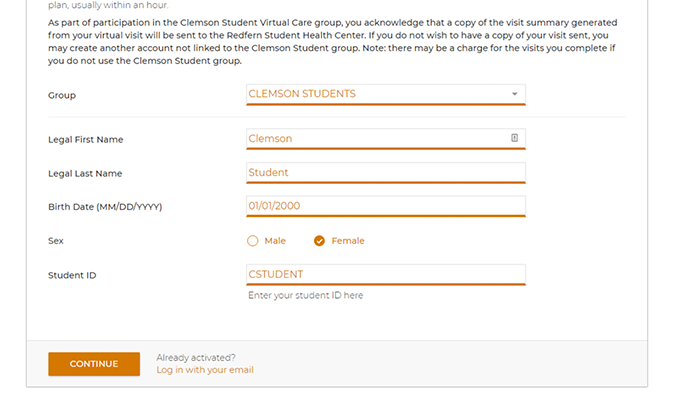This rectangular image is laid out with its long side extending horizontally from left to right, and appears to be a segment from either a website or app interface, albeit with its top and bottom sections slightly cut off. 

The image is bordered by a thin gray line, and a light gray banner runs across its bottom portion. Within this banner, there is an orange "Continue" button on the left side. To its right, a text prompt asks, "Already activated? Log in with your email."

At the top of the image, a detailed paragraph outlines that, as part of participating in the "Clemson Student Virtual Care Group," acknowledgment is required for a copy of the visit summary from virtual visits to be sent to the "Redfern Student Health Center." It specifies that if users prefer not to have their visit summaries sent, they may create an independent account not linked to the Clemson student group, though this might incur charges for completed visits.

Below this paragraph is a form. On the left side of the form are labels, and on the right are corresponding input fields pre-filled with information. They include:

- Group: Clemson students
- First Name: Clemson
- Last Name: Student
- Birth Date: 01-01-2000
- Sex: Male (unchecked), Female (checked)